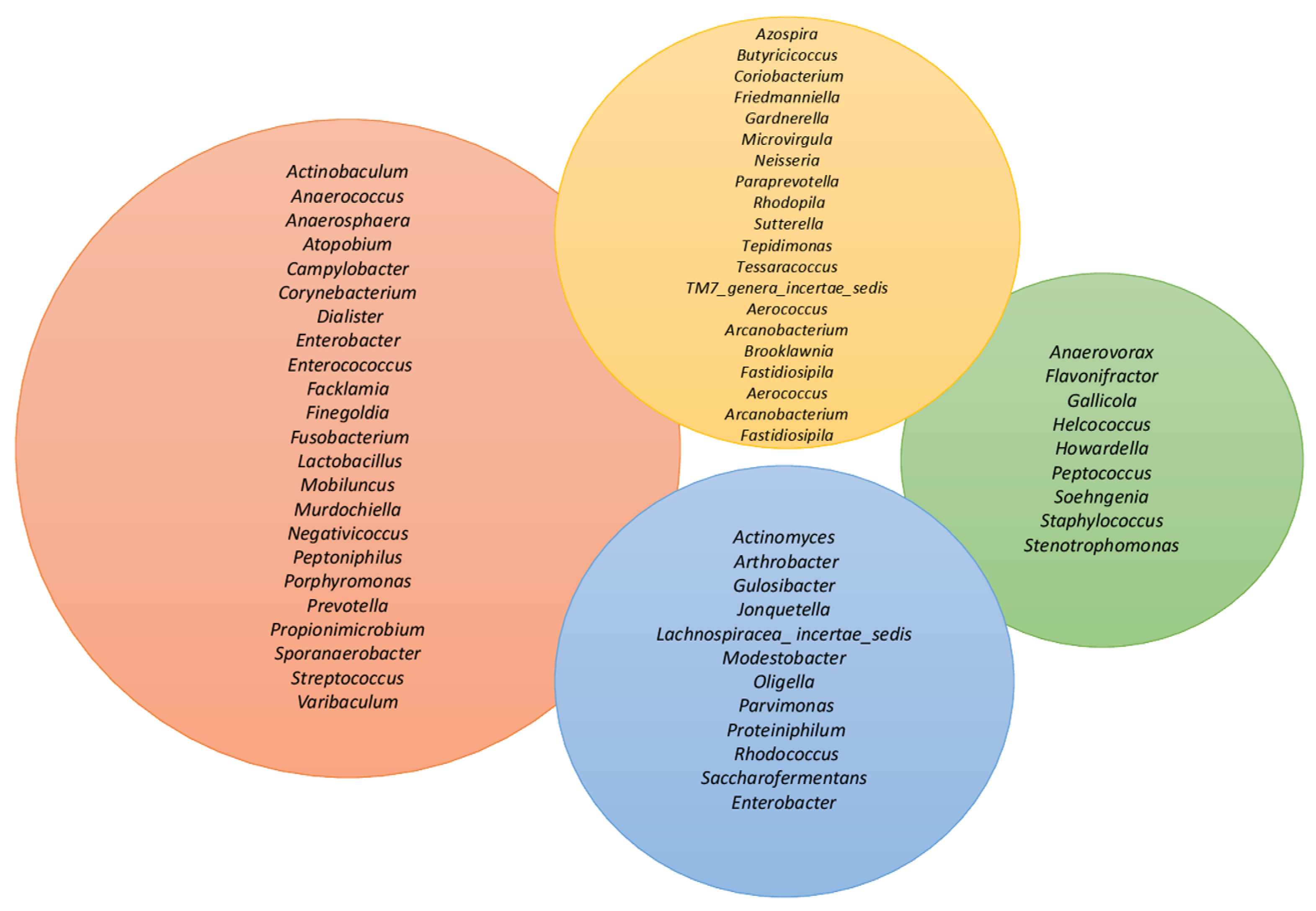This image, seemingly created using a computer program like Microsoft Word or PowerPoint, features four circles of varying sizes, each with detailed lists of complex, hard-to-pronounce bacterial names, center-aligned and arranged one word per line. On a clean white background, the largest and deepest circle, positioned on the left (or West), is a vibrant reddish-orange, containing the most extensive list. At the top (North) is a yellow circle, slightly smaller in size, also presenting a vertical list of bacterial names in black text. On the right (East), there's the smallest circle, colored green, with another list of terms. Finally, at the bottom (South), a bright blue circle, equal in size to the yellow one, contains a similarly lengthy list. Notable bacterial names across these circles include Acetonobacterium, Enterococcus, and Staphylococcus, distinguishing the array with some more recognizable names amid the largely foreign, intricate terminology.